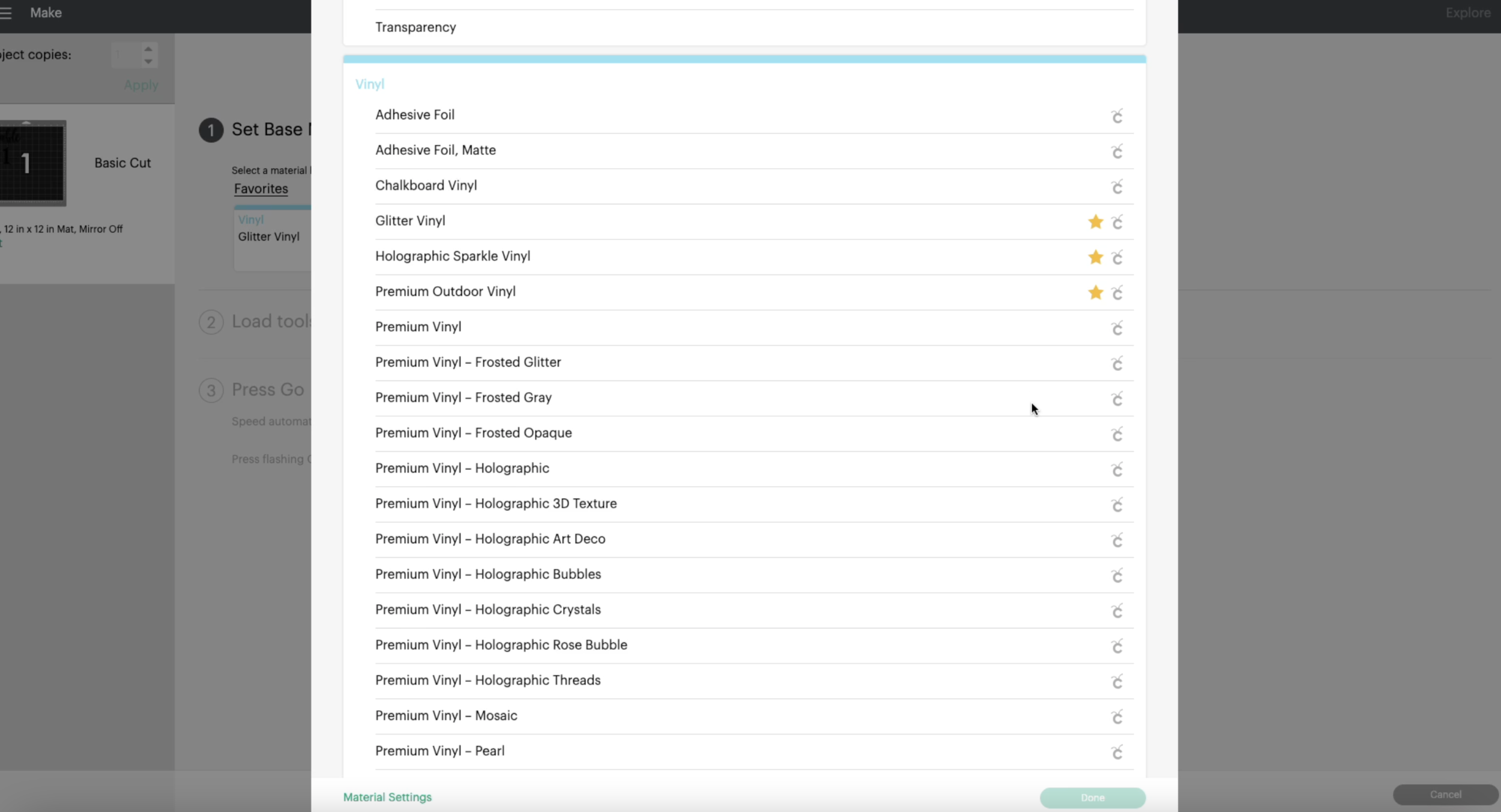The image is a screen capture taken from a desktop computer displaying an online application interface. The overall background of the displayed page is a light gray, with certain sections appearing grayed out. On the left side of the screen, two additional vertical frames or windows are also grayed out, blending into the background. Dominating the foreground is a large, prominent pop-up window with a clean, white background. 

At the very top of this pop-up, the word "Transparency" is written in bold, underscoring the focal point of the window. Directly beneath "Transparency," a vibrant blue horizontal line adds a dash of color and visual separation. Following this line, the word "VINYL" is written in all caps and spelled out phonetically as V-I-N-Y-L in a striking blue hue. 

Below this, a list of items is presented, each term arranged in a column and written in black. From top to bottom, the listed items include "adhesive foil," "adhesive foil mat," and "chalkboard veil." These words are clearly delineated, making it easy for the viewer to understand the contents and options available within this part of the online application.